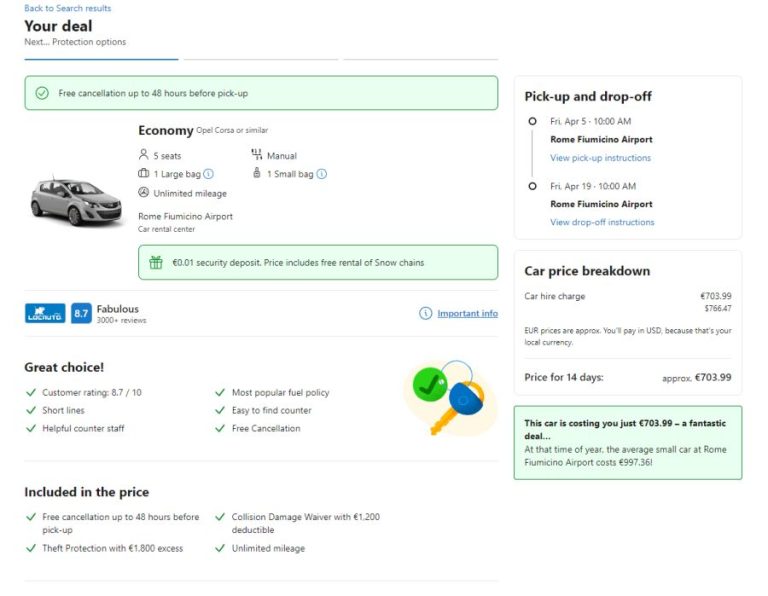This photo depicts a detailed search results page from a car rental website, captured in a square, portrait-oriented image against a white background. The page is bordered undefined, creating a seamless display. At the top, the page displays a blue heading reading "Search Results," followed by a black header stating "Your Deal." Below this, another header reads "Next Protection Options," with three spaced horizontal lines beneath—blue for the first line and gray for the subsequent two.

Further down, a green rectangular box with black text and a green check mark appears. This is followed by another header labeled "Economy," detailing an available car: "Opel, Corsair, or similar." Additional specifications include "five seats, one large bag, manual transmission, one small bag, unlimited mileage," and a mention of the "Rome Fremont Airport Car Rental Center."

A green box below states, "One euro security deposit price includes free rental of snow chains." Adjacent to this, a blue box with white text highlights an 8.7 rating labeled "fabulous." 

Under a thin gray border, the image showcases a "Great Choice" section supported by statistics in black text and marked by a green check mark. Finally, a section titled "Included in Price" is outlined, featuring two columns with rows of included amenities.